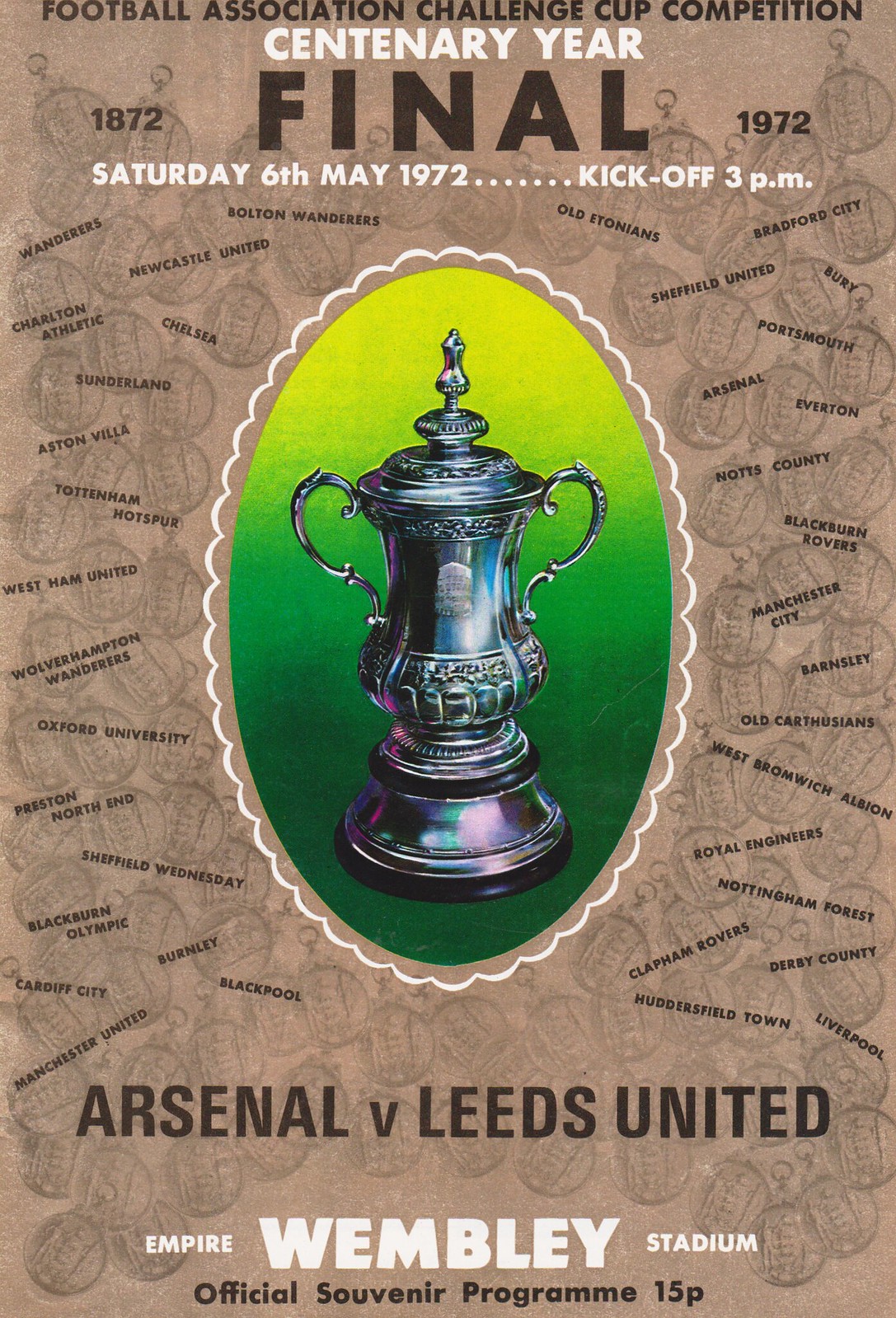This image is a detailed poster advertising a football event. The background is primarily light brown and covered with various small, coin-like awards. At the top, in distinct, bold black text, it reads "Football Association Challenge Cup Competition." Directly below in white text, it states "Centenary Year," flanked by the years "1872" on the left and "1972" on the right, with "Final" in bold black beneath that. Further details include the event date and time in white text: "Saturday, 6th May 1972... kickoff 3pm."

Dominating the center of the poster is an oval-shaped section with a green gradient background that transitions from dark to light green. In the middle of this oval is a prominent silver trophy cup, symbolizing the award for the competition.

At the bottom of the poster, large black text announces "Arsenal vs Leeds United," followed by a smaller white line detailing the venue: "Empire Wembley Stadium." Beneath that, in smaller dark brown text, it reads "Official Souvenir Program," with the price noted as "15p." Scattered throughout the background are the names of what appear to be players, completing the detailed and celebratory design of this centenary year final event poster.